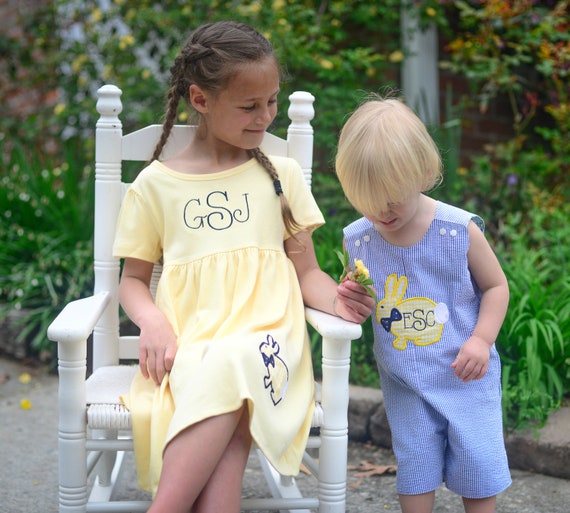This photograph, taken outdoors, captures a tender moment between two children standing on a concrete driveway. The focal point of the image is a young girl seated in a charming white wooden rocking chair positioned on the left. She has dark brown hair neatly braided into pigtails and is dressed in a bright yellow short-sleeved dress. Prominently displayed on the chest of her dress are the initials "GSJ" embroidered in blue, and near the bottom right, there's an intricate outline of a rabbit. She appears to be smiling gently as she looks at her younger brother and holds a yellow dandelion.

To her right stands a younger boy, a few years her junior, with light blonde bowl-cut hair. He is dressed in a blue and white striped one-piece outfit with overall shorts that are fastened by white buttons at the shoulders. Adorning the front of his outfit is a yellow rabbit with a blue bow tie and a small white tail, alongside the initials "ESC" in the center of the rabbit, mirroring the theme of his sister's dress. The boy is gazing down at the dandelion in his sister’s hand, seemingly fascinated by it.

Behind them, a concrete barrier serves as the boundary for a well-maintained flower bed filled with various green plants and shrubs, adding a touch of natural beauty to the scene. This harmonious blend of personal connection and the serene outdoor setting is captured in a square frame, presenting a wholesome and endearing glimpse into a moment shared between siblings.